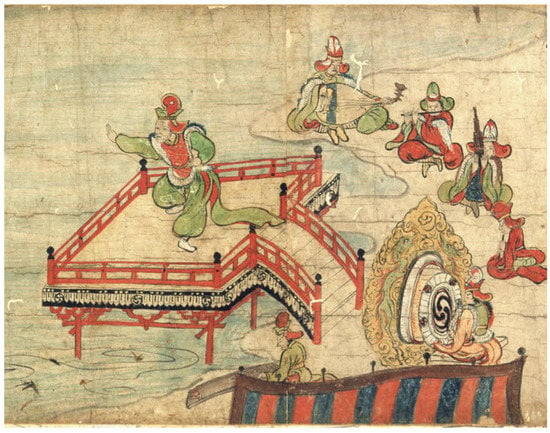In this detailed and intricately illustrated image, set against a light brown background with dark brown, curved lines suggesting the flow of water, we see a central platform raised on red legs. This platform, made distinct with red railings capped in black, is accessed by steps leading up from the ground. Atop the platform, which appears beige, stands a figure in a dynamic pose, possibly dancing or performing. The figure is dressed in flowing green garments, with notable red accents on the chest and head, giving the impression of movement and energy.

Surrounding this central action, the scene extends to the right where multiple figures—all in varied costumes and poses—are depicted. Among them, a man in a minimal green vest with a red hat stands firmly, holding what appears to be a large shield. Another figure nearby plays a flute, adding an auditory element to the visually rich scene. In total, there's a group of six individuals engaged in playing instruments, contributing to what seems to be a celebratory or ritualistic atmosphere.

The lower right corner features a patchwork of red and blue striped objects, further enhancing the scene's vibrancy. Collectively, the detailed costumes, the dynamic composition, and the engaging activities suggest this is an oriental-inspired artwork deeply rooted in cultural expression and artistic storytelling.